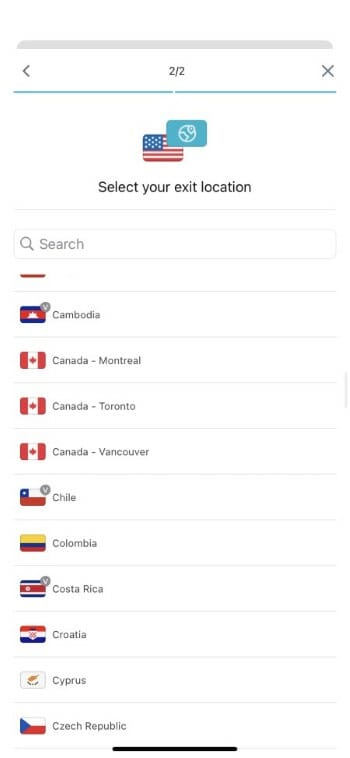The image depicts a mobile device displaying a particular app interface with a white background. At the top of the page is a thin gray bar with tabs; the open tab has a white background. On the upper left corner, there's a black back arrow. In the center, the numbers "2/2" are displayed. The top right corner features a black X. Below this section, there is an image of the American flag alongside a blue square containing a white globe icon. The text "Select your exit location" is prominently displayed underneath the icons, followed by a search bar. Below the search bar is a neatly organized list of countries and cities accompanied by their respective flags: Cambodia, Canada (with entries for Montreal, Toronto, and Vancouver), Chile, Colombia, Costa Rica, Croatia, Cyprus, and the Czech Republic.